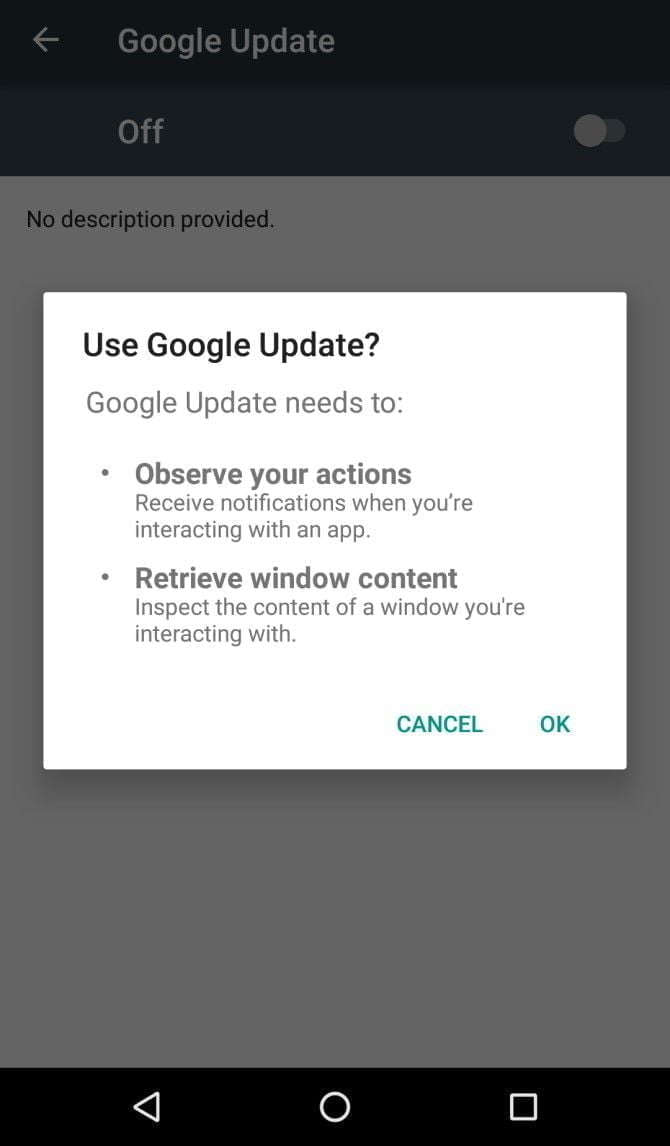This is a detailed screenshot captured on a cell phone displaying a notification pop-up with a white background and black text. The pop-up message reads, "Use Google update?" followed by "Google update needs to:" with two bullets underneath. The first bullet states "Observe your actions, receive notifications when you're interacting with an app," while the second bullet states "Retrieve window content, inspect the content of a window you're interacting with." The lower right corner of the pop-up features two functional links: "Cancel" and "OK," both highlighted in blue text.

In the background, the main page is dimmed with a dark overlay to emphasize the pop-up. At the top of this dimmed page, the title "Google update" is displayed with a left-facing arrow beside it, indicating a back navigation option. Directly below this title, there is a switch labeled "Off," which shows that the Google update feature is currently disabled. Beneath this switch, the text reads "No description provided."

At the very bottom of the screen, partially obscured by the pop-up, the standard navigation bar is visible with three icons: a left-facing arrow for back navigation on the left, a circular home button in the center, and a square icon on the right for accessing the overview of open apps.